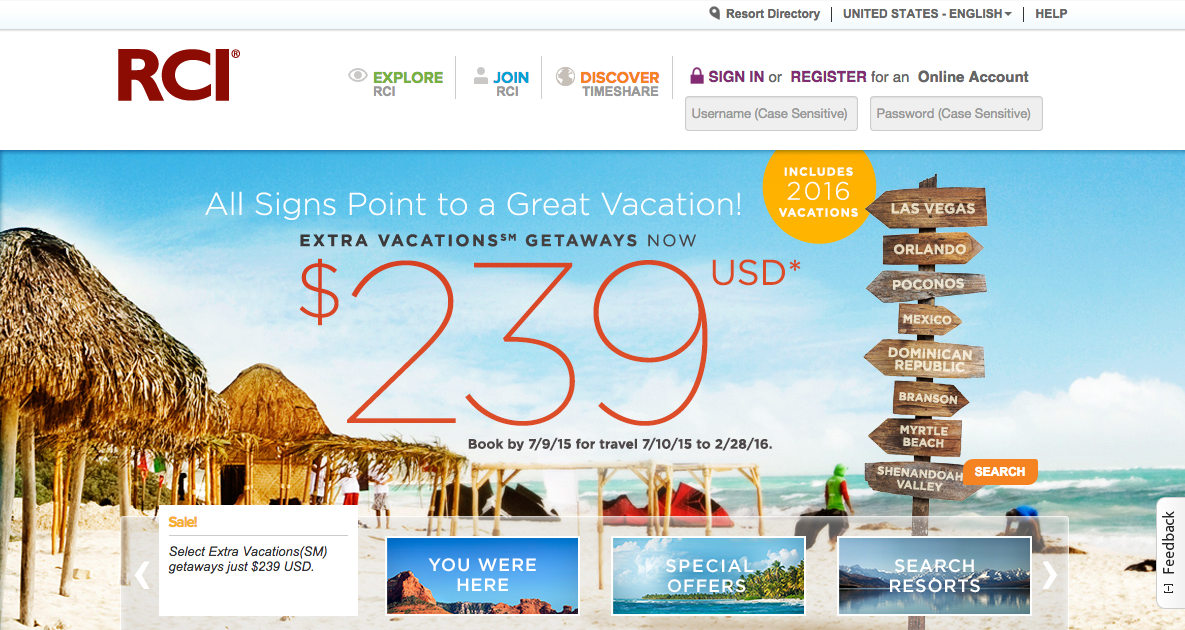The screenshot features a promotional webpage for a timeshare company, prominently displaying various interactive elements and offers. In the center, a vibrant image of beach huts is overlaid with several calls to action: "Explore" in green, "Join" in blue, "Discover" in orange, and "Sign In or Register" in purple. The top navigation bar includes options such as "Resort Directory," "United States," "English," and "Help."

Two gray rectangles at the top right prompt users for a "Username (case sensitive)" and "Password (case sensitive)," emphasizing account access for personalized experiences. Below, a striking red banner advertises a limited-time offer, "All signs point to a great vacation," highlighting "Extra Vacations Getaways" priced at "239 USD." A yellow circle notes that the promotion includes 2016 vacations, with a booking deadline of "7/9/15" for travel between "7/10/15" and "2/28/16."

At the bottom, three rectangular buttons offer navigation options: "You Were Here," "Special Offers," and "Search Resorts." Lastly, a "Feedback" link is positioned to the right, encouraging user interaction and website improvement suggestions. The overall design suggests an enticing and organized layout tailored for enhancing user engagement and driving bookings.